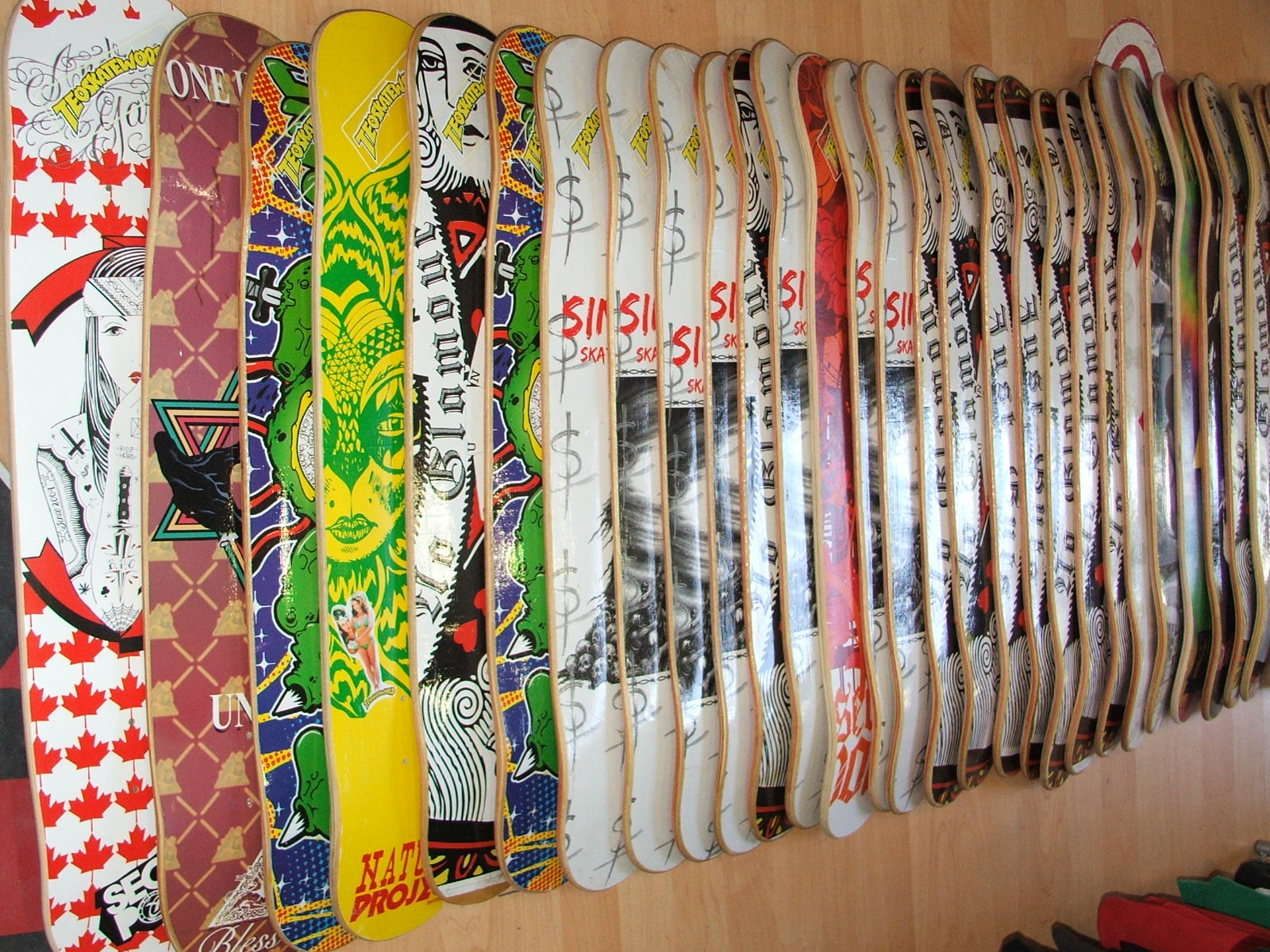The color photograph depicts the interior of a skate shop with a light-colored wood-paneled wall. The wall is adorned with a single row of overlapping skateboards, each without wheels or trucks. The skateboards are mounted horizontally, creating a visually engaging and colorful display. On the far left, one skateboard is prominently decorated with red Canadian maple leaves and features a cartoon-like female figure in the center. Numerous other boards overlap like a cascade of band-aids, each showcasing distinct graphic designs, logos, and sponsor images. Among them, a yellow board with a green jester face and another set of white boards marked with black dollar signs can be seen. The overall display illustrates a variety of colors and patterns, emphasizing the vibrant and diverse designs typical in skateboarding culture. In the bottom right corner, there are some red and green objects on the floor, resembling shoes—possibly skateboarding shoes like Vans—or other skateboarding accessories.